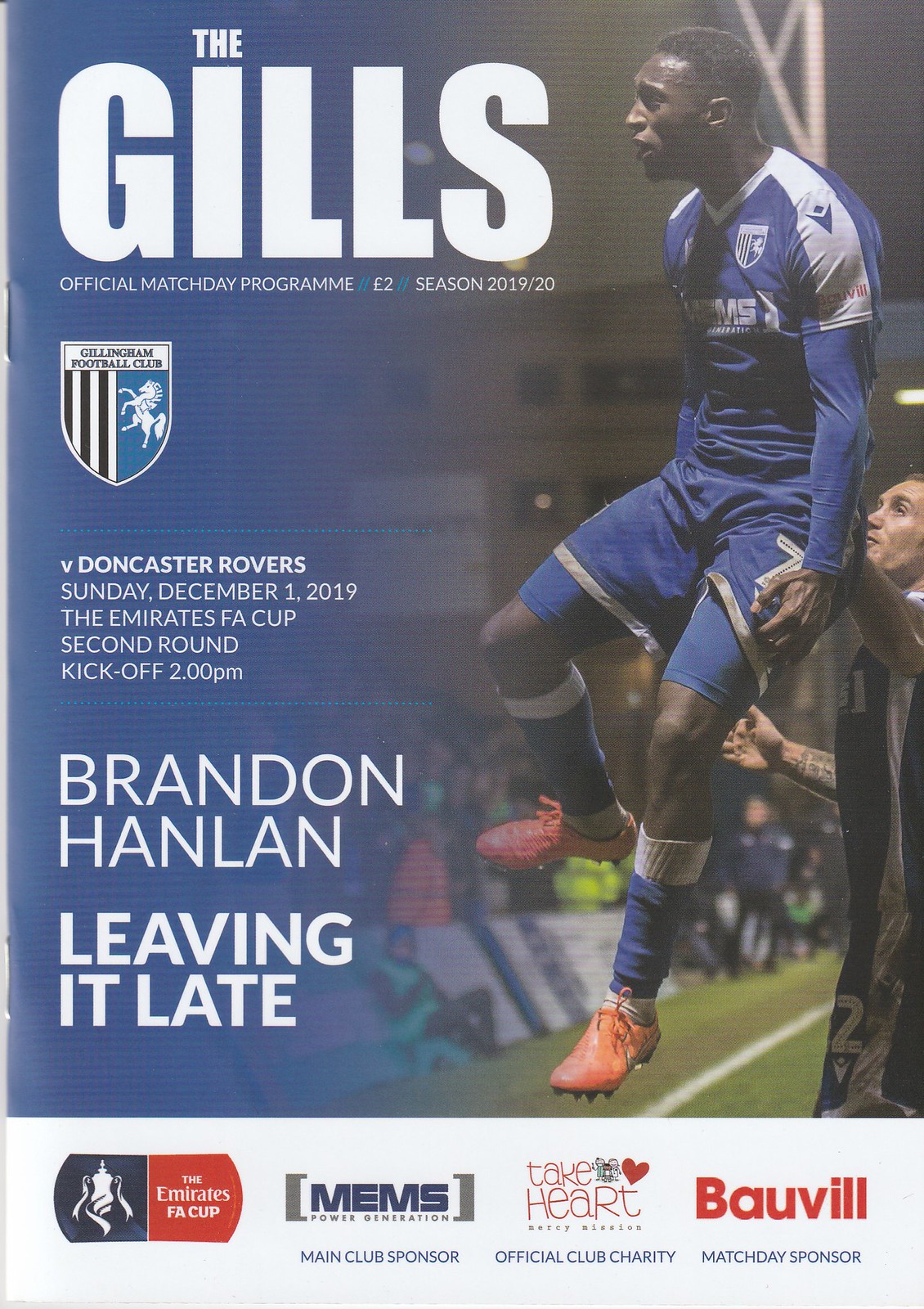The cover of the magazine prominently features a dynamic photograph of Brandon Hanlon, a black soccer player, soaring impressively high into the air, his waist aligning with the head of a defender behind him. He is wearing orange soccer cleats with black bottoms, tall blue socks with white knitted tops, blue shorts with silver hems, and a short-sleeve blue soccer jersey with white stripes along the sleeves and around the collar. Positioned in the background, another player is seen wearing a nearly identical uniform. To the left of this action-packed image, there is text in white that reads: "The Gills Official Match Day Program £2 Season 2019-20." Below this, the Gillingham Football Club’s black and white vertically striped shield with a horse emblem is displayed, alongside details of the match: "Gillingham Football Club versus Doncaster Rovers, Sunday December 1st, 2019, the Emirates FA Cup Second Round, kickoff 2 p.m." Additionally, the left side of the cover also features the text "Brandon Hanlon Leaving It Late" further highlighting the key player. At the bottom, it notes, "The Emirates FA Cup MEMS Main Club Soccer Take Heart Official Club Charity Ball Bill Match Day Sponsor."